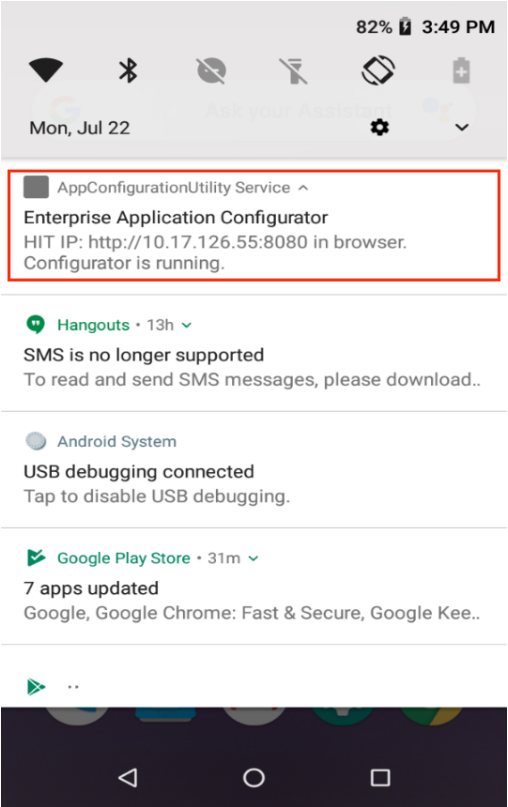The image is a detailed screenshot of a cell phone screen, roughly twice as tall as it is wide. In the upper right corner, the battery icon shows 82% with a lightning bolt, indicating the phone is currently charging. The time displayed next to the battery icon reads 3:49 PM.

In the top section of the image, there are various menu options on the left. These include icons for Wi-Fi, Bluetooth, a circle with a minus sign (which could signify "Do Not Disturb" mode), a flashlight icon with a slash through it (indicating it is turned off), a vibrate icon, and a power icon.

Below these options, the date is shown: "Monday, July 22nd." Adjacent to the date, there is a settings icon (represented by a gear) accompanied by a black down arrow.

The central part of the screen has a white background with the title "App Configuration Utility Service" at the top. Following this title is an upward arrow. Underneath, in bold black text, it says "Enterprise App Application Configurator." Further down, in gray text, there's the heading "IP Address," followed by a specific IP address (which isn't fully visible in the description), and the phrase "in browser."

At the bottom of this section, "Configurator is running" is highlighted with a red rectangle, drawing attention to the notice. Below this, a message indicates that "Hangouts SMS is no longer supported."

Every detail on the screen is clearly depicted, emphasizing various functionalities and notifications available to the user.